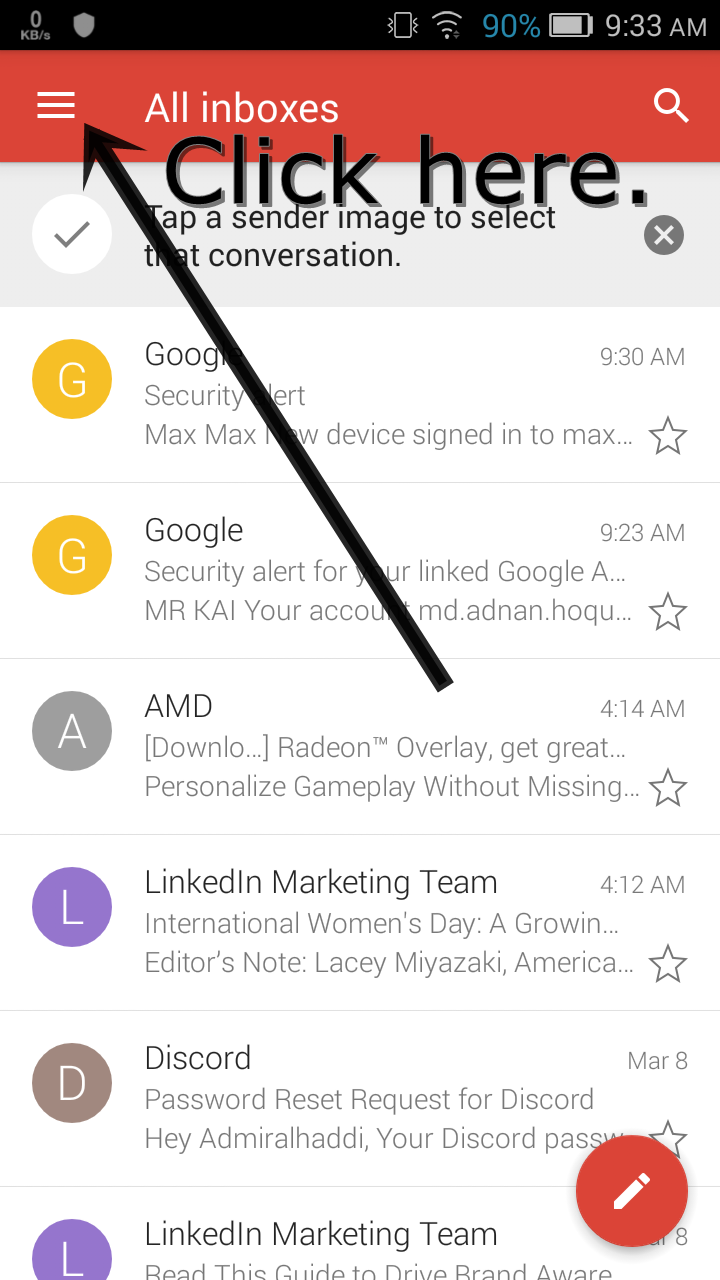The screenshot captures the interface of a mobile phone displayed in portrait orientation. At the very top of the screen is a horizontal black bar that houses several elements in white: on the left, it reads "0 KBs" adjacent to a light gray shield icon. On the right side are several white icons, including indicators for a ringer (showing it is active), Wi-Fi signal strength, and a battery icon accompanied by "90%" in blue text. The time is displayed as "9:33 AM" on the far right.

Below this is a wider red horizontal bar, featuring three horizontal white lines on the upper left (a common symbol for a menu), and a central black arrow pointing diagonally from the bottom of the image towards the menu icon. Centrally placed in this bar is the text "All Inboxes" in white, and a white magnifying glass icon is situated on the far right. Superimposed on this red bar and extending slightly into the white background below are large, bold black letters spelling "Click Here," which seem to correlate with the arrow.

Underneath, there is a text line instructing, "Tap a sender image to select that conversation." To the left of this instruction is a white circle with a black checkmark, and on the right is a gray circle with a white "X."

The main section of the screen displays six rows of listings. The details are as follows:

1. The first listing has a mustard-colored circle with a white "G" on the left, indicating a Google-related alert. The text reads, "Google Security Alert, Max Max Low Device signed into Max," with a star icon on the right.
2. The second line, also marked by a mustard circle with a white "G," reads, "Google Security Alert for your linked Google account, Mr. Kai, your account, MD, Adnan, Hulk," which truncates with three horizontal black dots and ends with a black star.
3. The third listing features a gray circle on the left with a white capital "A," and the bold text "AMD." It mentions "Radeon overlay, get great" and "Personalize gameplay without missing," both of which are cut off, and has a star icon on the far right.
4. The fourth row depicts a purple circle with a white "L," labeled "LinkedIn Marketing Team," discussing "International Woman's Day," and has a star icon on the right.
5. The fifth entry displays an off-color gray circle with a white "D," reading "Discord, password reset request for Discord."
6. The sixth and final line shows a purple circle with a white capital "L," denoting another message from the LinkedIn Marketing Team. The text "Read this guide to drive brand aware" is cut off, and on the right, there is a large red circle with a white diagonal pencil icon.

Overall, the image portrays a phone screen showing multiple notification alerts from various applications and services, providing a snapshot of the device's current active notifications and interface elements.